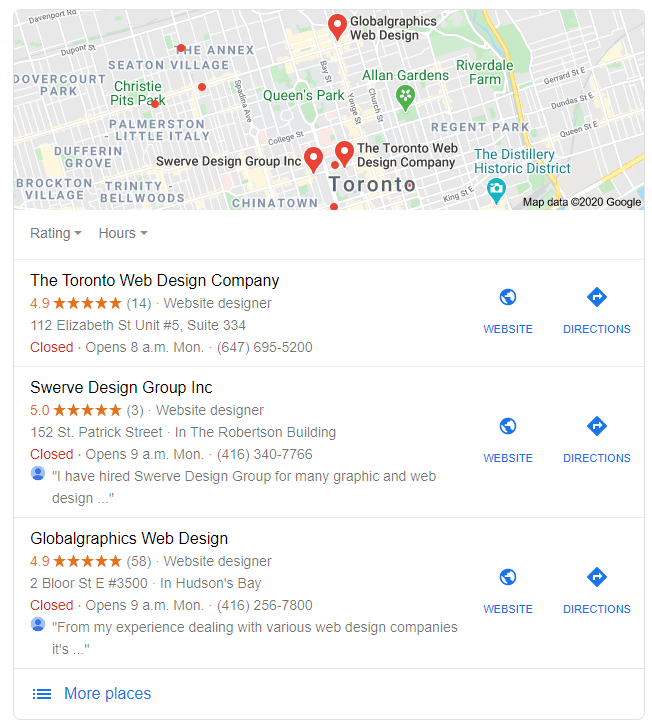**Caption:**

The image features a detailed map with direction information and relevant details. The map is color-coded in shades of gray, green, yellow, and black, highlighting various notable areas in Toronto such as Christie Pits Park, Queen's Park, Allan Gardens, Riverdale Farm, Regent Park, and The Distillery Historic District. Prominently labeled "Toronto" appears in bold on the map. Below the map, there are filters for rating and hours.

Listed below are several web design companies with detailed information:

1. **Toronto Web Design Company**
   - Rating: 4.9 stars (14 reviews)
   - Type: Website Designer
   - Address: 112 Elizabeth Street, Unit #5, Suite 334
   - Status: Closed, opens at 8 a.m. on Monday
   - Contact: 647-695-5200
   - Additional: Website and directions available

2. **Swerve Design Group Inc.**
   - Rating: 5 stars (3 reviews)
   - Type: Website Designer
   - Address: 152 South Patrick Street, Robertson Building
   - Status: Closed, opens at 9 a.m. on Monday
   - Contact: 416-340-7766
   - Additional: Endorsed for graphic and web design services

3. **Global Graphics Web Design**
   - Rating: 4.9 stars (58 reviews)
   - Type: Web Designer
   - Address: 2 Bloor Street East, Suite 3500, Hudson Bay
   - Status: Closed, opens at 9 a.m. on Monday
   - Contact: 416-256-7800

Additional places and contact details are seen below, along with 'website' and 'directions' links on the right-hand side of the image.